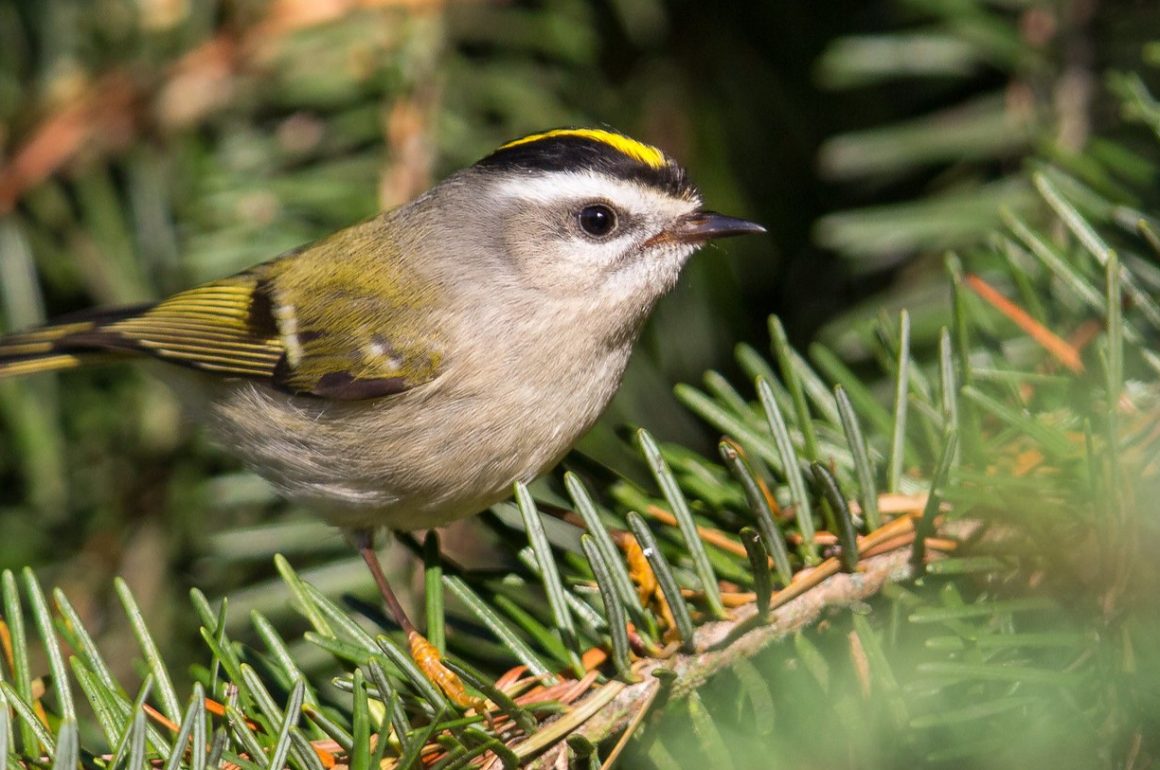A color photograph depicting a small, chubby bird perched on a brown branch of a pine tree with thin, green needles. The lifelike but possibly computer-generated image shows intricate details of the bird, which has a beady black eye, a small black and brown beak, and rounded features. The bird's plumage is primarily gray and light brown, with a pale gray chest. Its head is adorned with black feathers and a bright yellow stripe, complemented by white striping around its eye. The wings and tail feature a mixture of yellow and dark brown highlights. The background is blurry, bringing the focus to the bird and the pine tree branch, which despite its artificial appearance, adds a naturalistic touch to the scene.